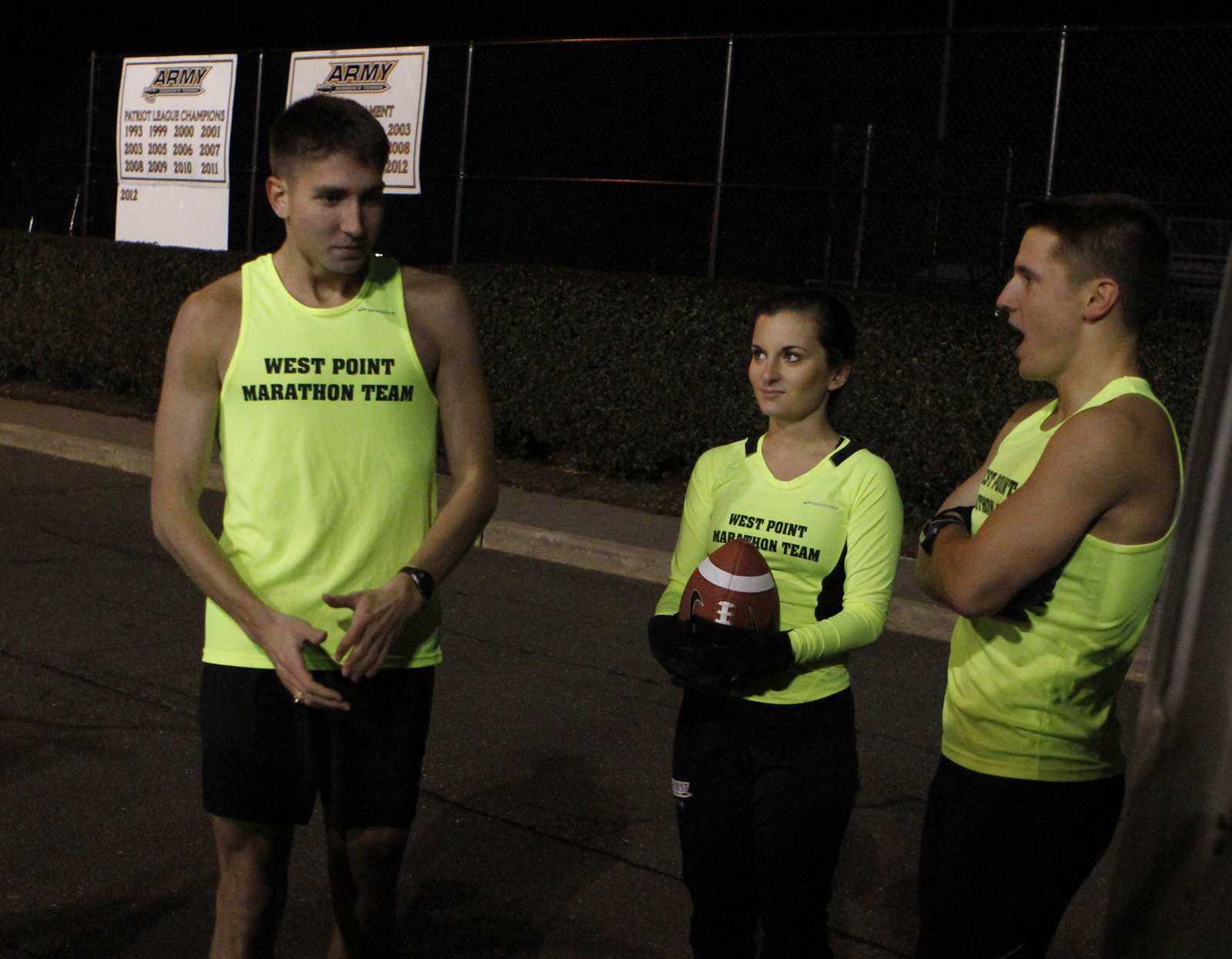In this indoor setting, a photograph captures three West Point cadets standing side by side with a darker background. The two men are wearing yellow tank tops emblazoned with "West Point Marathon Team" in black letters, while the woman at the center sports a matching long-sleeve green jersey. All three are dressed in shorts, with the men also wearing black wristwatches. The woman, who stands slightly shorter than the men, is holding a football and looking upward toward the taller man on her left. Behind them, a shelf and wall are visible, decorated with two white signs that read "Army" and list the years from 1993 to 2012, indicating Patriot League Championship victories. The setting suggests a strong affiliation with West Point and its athletic achievements.